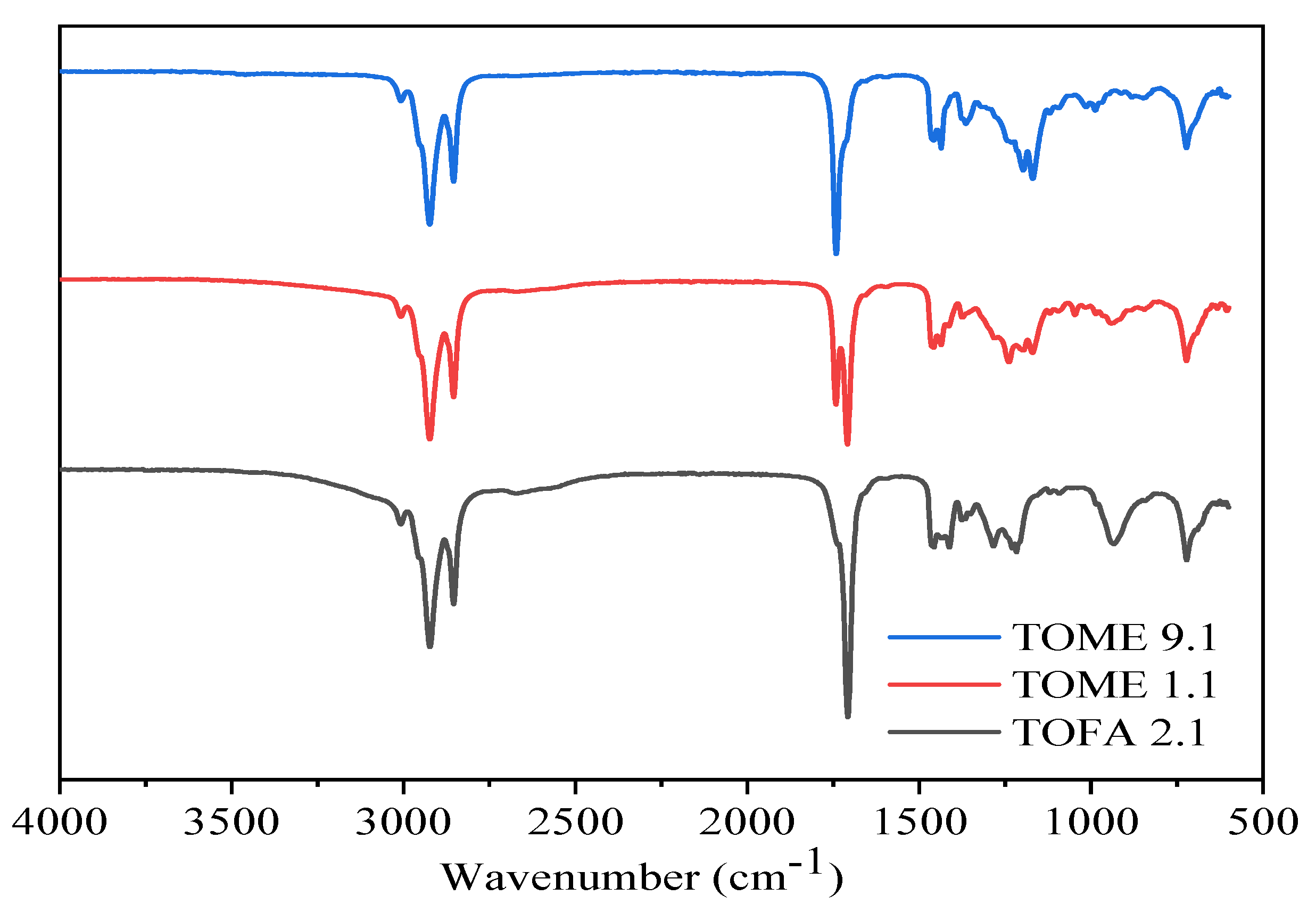The image presents a detailed chart depicting a photocatalysis spectrum, characterized by an IR spectrum plot within a rectangular black background. The graph features three distinct lines, each with a series of peaks and valleys, resembling an electrocardiogram (EKG). The top line in blue, labeled as TOME 9.1, is followed by a middle red line labeled TOME 1.1, and a bottom grayish-black line labeled TOFA 2.1. These lines are plotted against an x-axis that measures wave number in centimeters to the power of minus one (cm⁻¹), ranging from 4,000 to 500. Specific markings on this axis include 4,000, 3,500, 3,000, 2,500, 2,000, 1,500, indicating various critical points of measurement. The lines, while mostly parallel, exhibit slight differences and share common features, such as two deep valleys toward the end, which culminate in an erratic pattern.